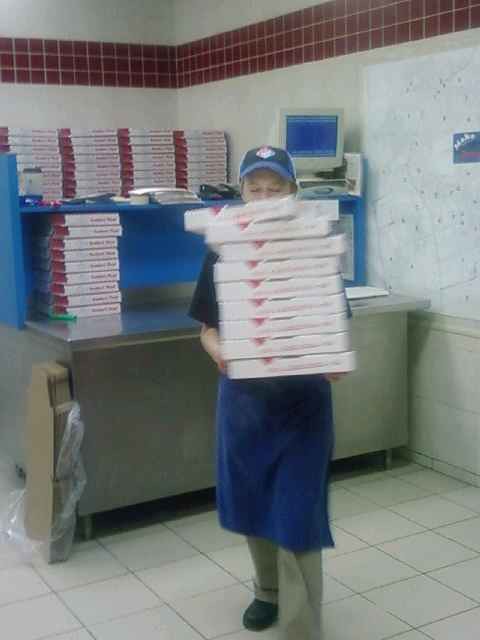In this dynamic scene from a bustling pizza takeaway business, a dedicated employee is captured mid-shift, securely balancing a stack of nine pizza boxes. She is dressed in a long blue apron over a black t-shirt and light green khakis, complemented by black shoes. A blue baseball cap with a logo sits on her head, indicating the company's branding. The backdrop of the image reveals a stainless steel workbench topped with an old-fashioned computer displaying a blue screen with text, and cluttered with scattered pieces of paper. Multiple stacks of white pizza boxes, each marked with a dark red slot for identification, are neatly organized behind her, some on the floor and others on the table. To the left, unfolded brown boxes are ready to be assembled into more pizza containers. The room itself features beige or off-white walls adorned with a decorative strip of dark red tiles near the ceiling, enhancing the functional yet busy atmosphere of the pizza place.